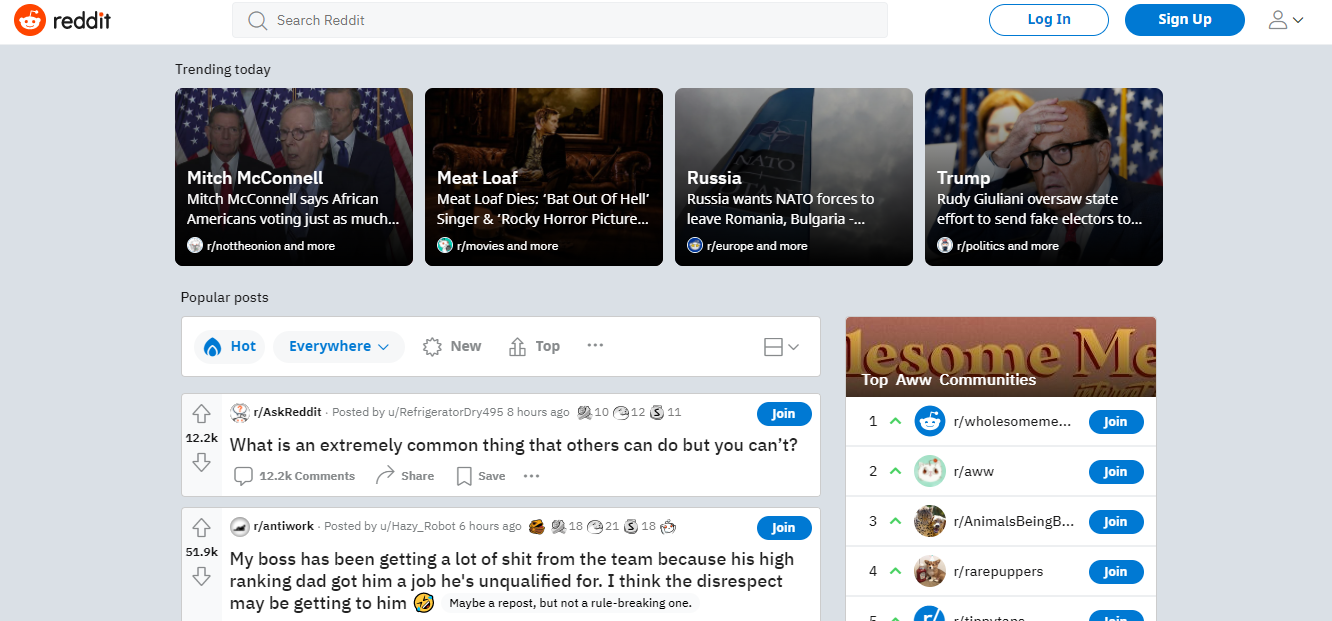At the top of the image, there's a prominent Reddit emblem accompanied by the word "Reddit" adjacent to it. Moving horizontally from left to right, the header includes options such as "Search Reddit," "Login," and "Sign Up." Beneath this header, a gray rectangle spans the width, containing four black boxes. Each box houses a photo with a caption. The first box is titled "Trending Today" and showcases the current trending topics: Mitch McConnell, Meatloaf, Russia, and Trump.

Below this section, there are three white rectangles. The first rectangle features navigation options: "Hot," "Everywhere," "New," and "Top." The second rectangle displays a question, "What is an extremely common thing that others can do but you can't?" alongside a blue "Join" button. Directly underneath, another entry reads, "My boss has been getting a lot of SHIT from the team because his high ranking dad got him a job he's unqualified for. I think the disrespect may be getting to him." This is accompanied by a sideways laughing face emoji and another blue "Join" button.

To the right of these rectangles, there's a burgundy box with partially visible yellow lettering that spells out "L-E-S-O-M-E," followed by "M-E," with the full word not entirely visible. Additionally, five join buttons are aligned on the right side, each next to small round emblems on the left, interspersed with black-lettered words in between.